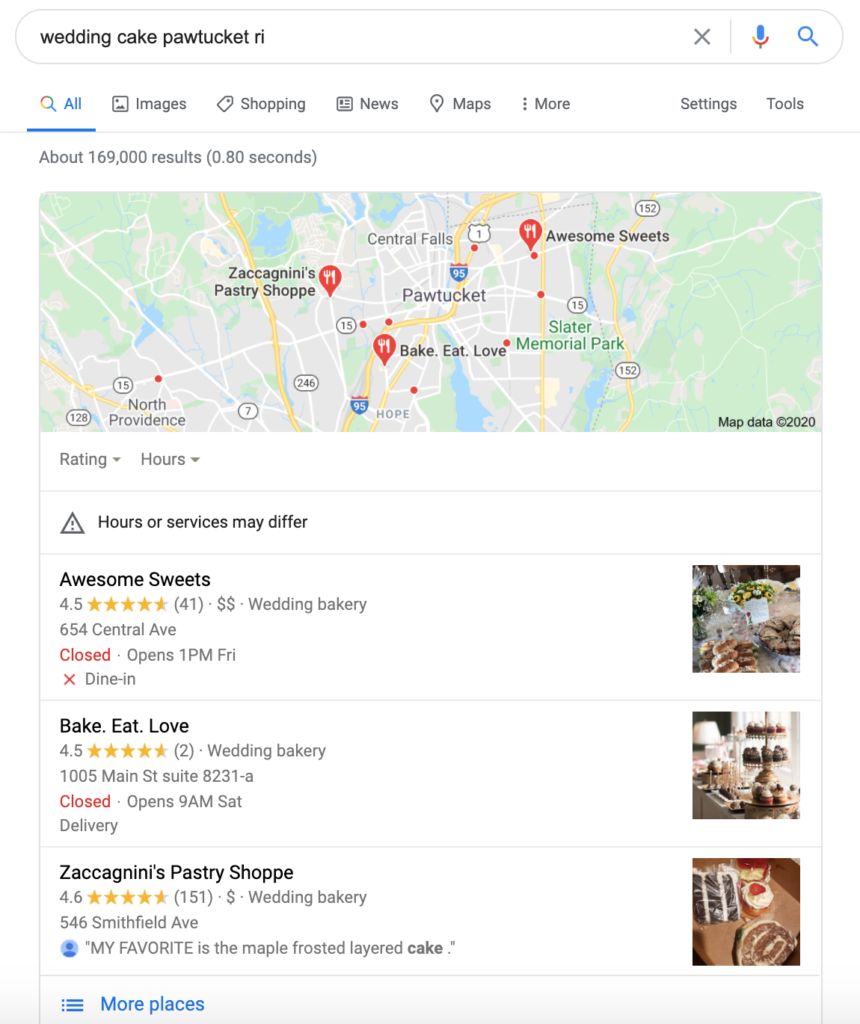A detailed caption for the given image could be:

"This image captures a Google Maps search results page focused on 'Wedding Cake,' specifically in Pawtucket, Rhode Island. The top of the screen displays the search query in the search bar: 'Wedding Cake, Pawtucket, R.I.' Underneath, the 'All' tab is highlighted in blue, indicating that it's showing all relevant results. The central portion of the map highlights Pawtucket with three specific pastry shops pinned: 'Awesome Streets' to the right, 'Bake Eat Love' to the bottom-left, and 'Zach Agnes Pastry Shop' also to the left of Pawtucket's center. Below the map, a list of these locations is displayed, accompanied by thumbnail images of the pastry shops, showing a variety of stacked pastries. Each listing boasts a five-star rating. Notably, the top two shops appear to be currently closed, while the third listing, Zach Agnes Pastry Shop, features a positive quote: 'My favorite is the maple frosted layered cake.' At the bottom of the screen, there is a clickable option labeled 'More places' in blue, inviting users to explore additional results."